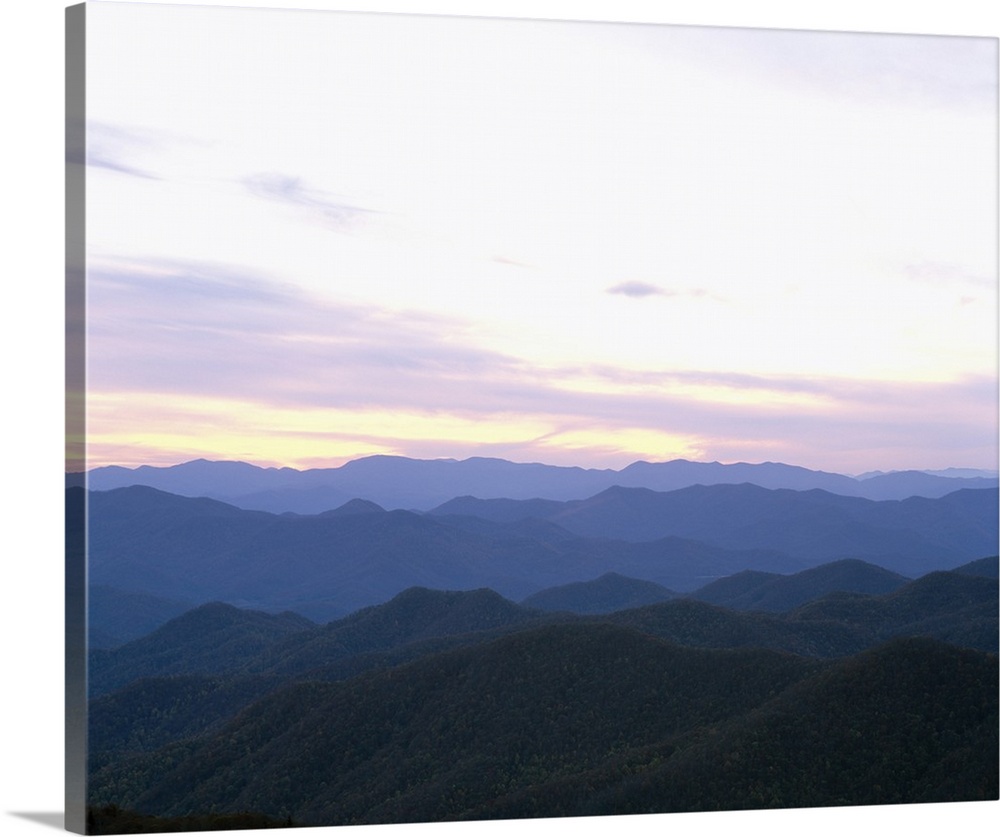This captivating artwork showcases a magnificent vista of undulating mountaintops extending into the distance. The painting skillfully employs various shades of blue and gray to differentiate the mountain ranges, creating a mesmerizing gradient from dark tones in the foreground to lighter tones as the eyes travel farther into the scene. At the lower part of the image, the mountains are almost black, transitioning to blue-gray and lighter blue-gray hues further back. The peaks, devoid of snow, appear brown and gray, contributing to the natural and rugged charm of the landscape.

Above the mountains, the sky is an overcast canopy adorned with multiple layers of clouds, subtly expressing tones of plum, light pink, and purples. Near the horizon or just behind a cloud bank, a faint yellow glow from the sun either setting or rising imbues the scene with a soft warmth, casting a serene glow across the expansive skyline. This intricate interplay of colors and light masterfully captures the tranquility and grandeur of the scene, inviting viewers to lose themselves in the never-ending rows of mountains and the serene beauty of this majestic panorama.